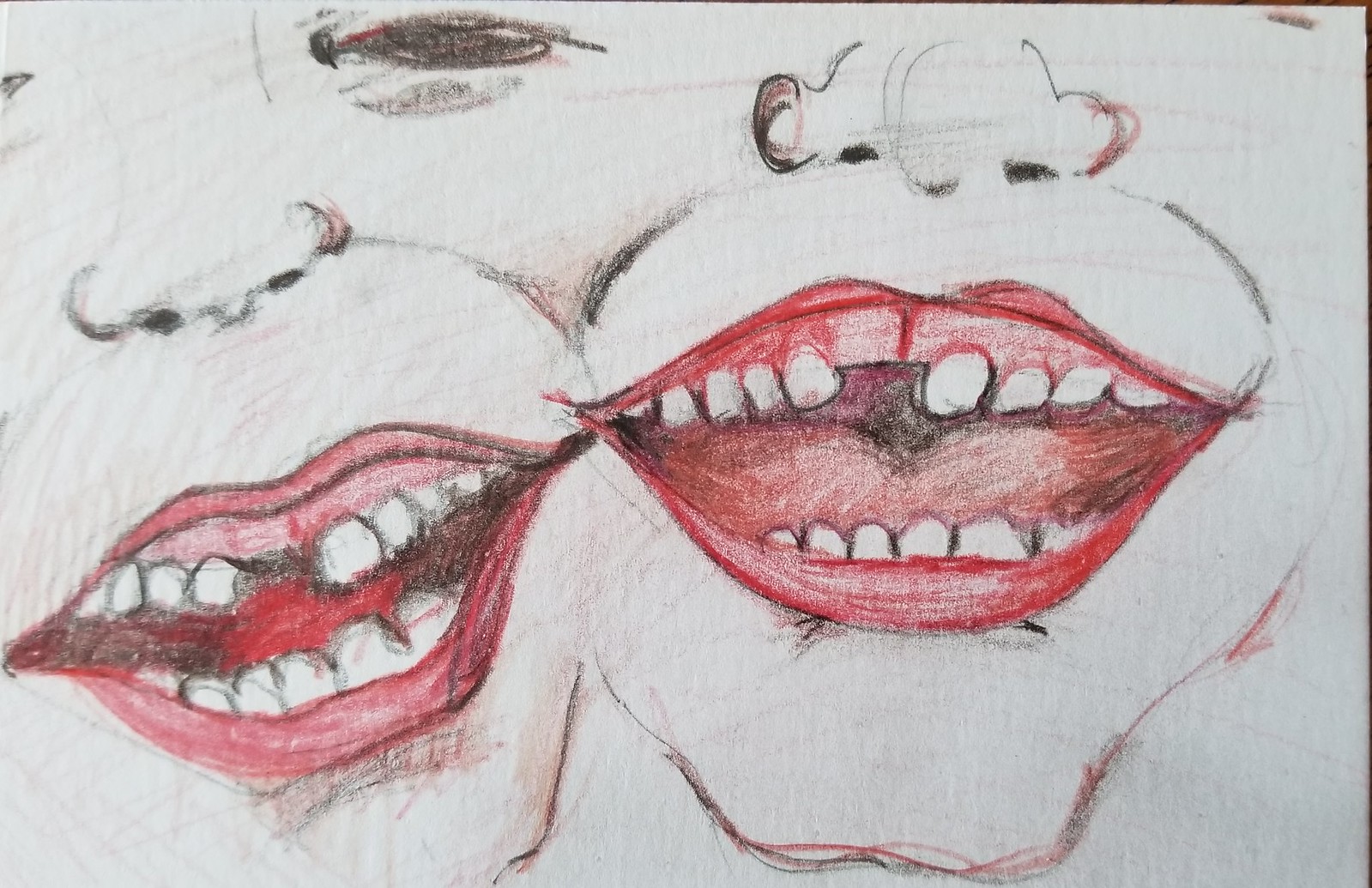The artwork is a colored pencil and charcoal drawing on paper, showcasing two abstract faces positioned side by side. The primary focus of the piece is on the mouth and nose areas of the faces. Both faces feature wide, vivid red mouths with the gums and lips also rendered in a bold, almost garish red. Each face displays white, gravestone-shaped teeth, with a conspicuous center gap and a missing left front tooth.

The eyes are particularly striking, characterized by all-black pupils that add a haunting quality to the expressions. Both faces have large, broad noses and asymmetrical, open mouths, giving them an exaggerated and somewhat unsettling appearance. Their chins are angular, with a subtle cleft, contributing to the abstract and stylized nature of the piece.

The overall composition is primarily white with black details, except for the vivid red accents on the mouths and a few red line highlights elsewhere, enhancing the dramatic effect. The imagery recalls the unsettling and exaggerated features of caricatures, making a bold and provocative visual statement.